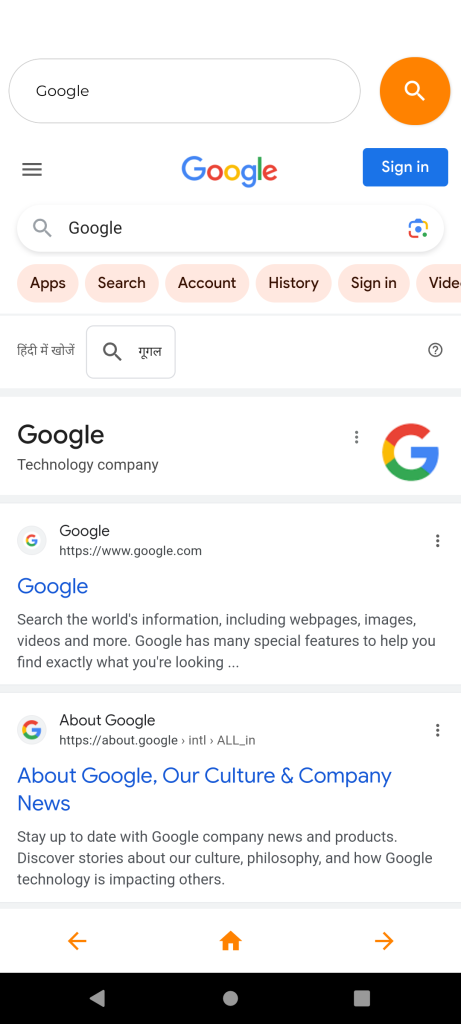The image appears to be a screenshot from what seems like the Google app on a cell phone. At the top, there is a prominent rounded-edge oval, which initially appears to be a search bar but may actually be the address bar. Within this oval, the word "Google" is displayed inside a large rectangle. There is an orange circle containing a white magnifying glass icon. Directly underneath, the well-known colorful Google logo is visible. Next to it, in a blue rectangle with white text, it says "Sign in." On the left side of this line, there are three horizontal bars.

Below this, there is a search window with a gray magnifying glass icon beside the word "Google" in black font. Adjacent to this, there is a camera icon in Google colors. 

Further down, there are six circles in a light orange hue, each containing a word in black font: "Apps," "Search," "Account," "History," "Sign in," and "Video" (with the 'O' partially cut off). There also appears to be Arabic text beneath these circles that translates to "Google, a technology company," followed by a description indicating "Google search the world's information including websites, pages." 

At the bottom of the image, there are three orange icons—a left-facing arrow, a house, and a right-facing arrow, suggesting navigation options within the Google app.